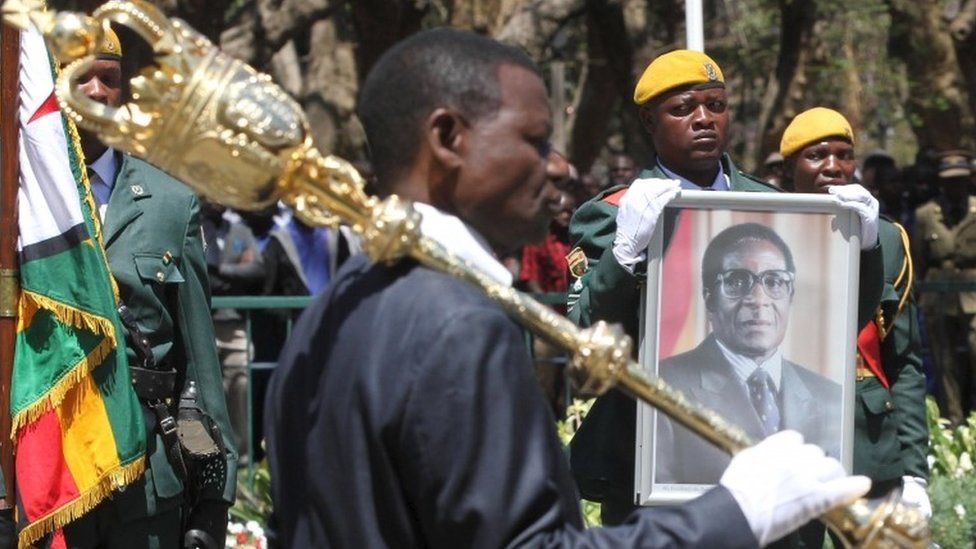This image captures a ceremonial or memorial service set against a rocky or forested backdrop. At the center stands a dignified black man in a shiny navy suit, wearing white gloves and holding a gold scepter adorned with an ornate royal crown-like symbol. He is oriented to the right, revealing his profile. Behind him, two men in green uniforms with blue shirts and yellow berets also wear white gloves. One of these men holds a large portrait of a bespectacled man in a gray suit and tie, likely a political figure. The expressions on their faces convey a serious, possibly somber mood. To the left, another man in a similar uniform holds a flag that features red, yellow, and green stripes with a cascading design, partially obscuring a detailed emblem in the center, framed by gold fringe. Just behind these focal figures are additional spectators and the indistinct outlines of a mountainous or forested terrain. The emphasis of the image is on the memorial nature of the gathering and the solemnity of the individuals involved.